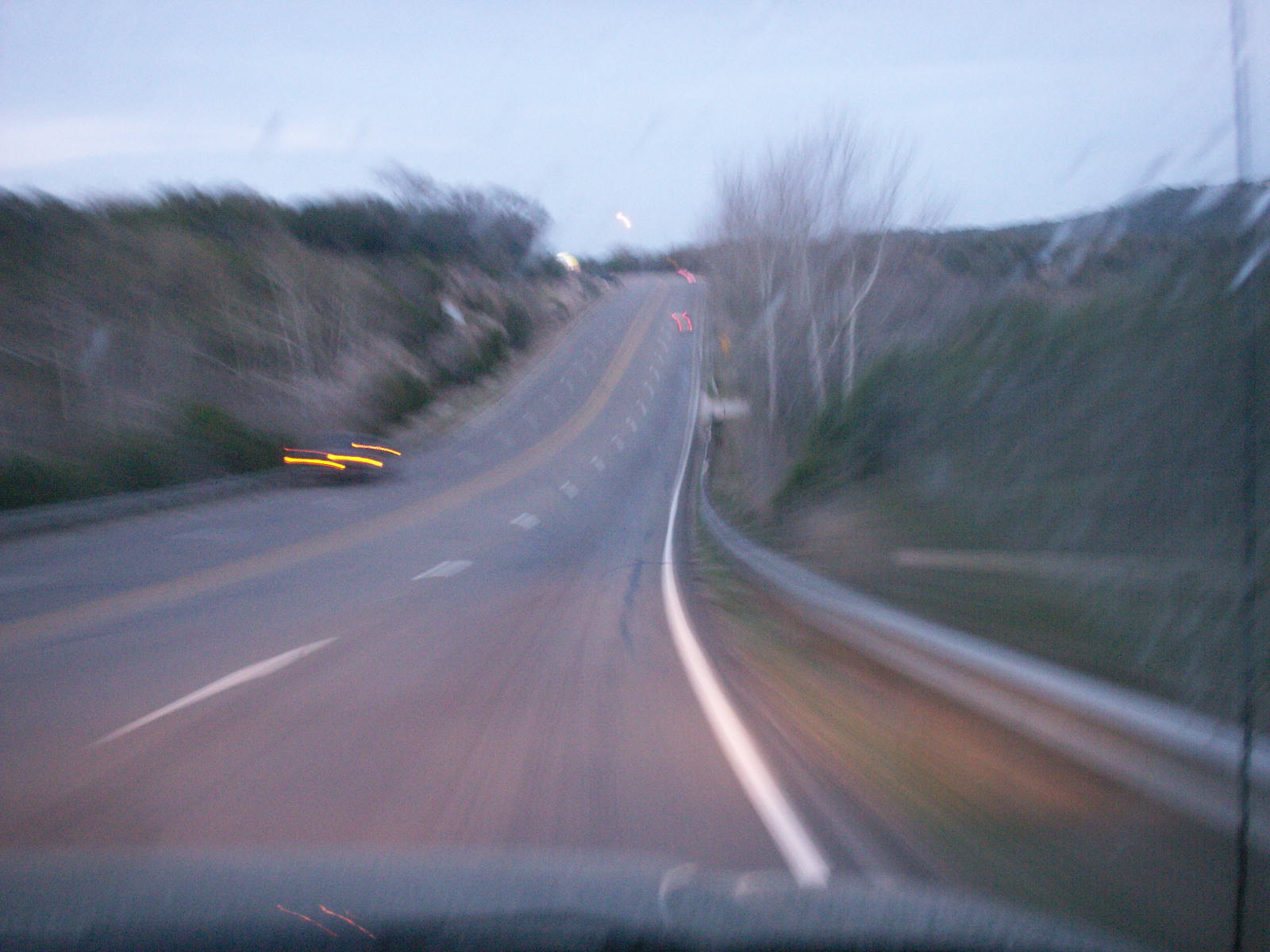A blurred image captures the view from inside a moving vehicle on a four-lane highway. The roadway is divided by a solid yellow double line in the center, with an additional set of lanes running parallel. A metal barrier lines the right side of the highway, separating it from a dense area of trees and grass. Farther ahead, the faint lights of an approaching car are visible through the motion blur. In the distance, the highway curves slightly upward, marked by the dim presence of brake lights from vehicles further along. The scene exudes a sense of desolation, accentuated by the sparse traffic and the encroaching wilderness.